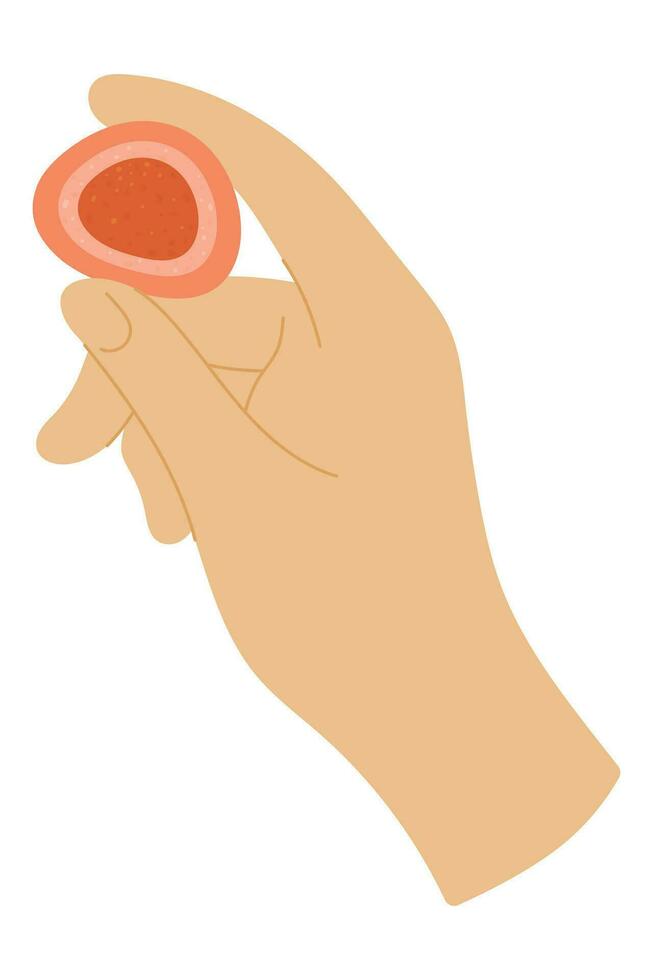This is a minimalistic cartoon illustration depicting a hand holding an ambiguous object, possibly a food item like Japanese mochi or a piece of fruit. The hand, drawn in light peach or beige tones with simple lines for the fingers and nails, suggests a Caucasian complexion. The object held is an oval or lumpy circle with a multilayered structure: an outer layer in a pinkish or orange hue, a middle light pink layer, and a central dark red or brownish circle. The object is also adorned with tiny yellow speckles. The image is set against a stark white background, with no additional elements or text.